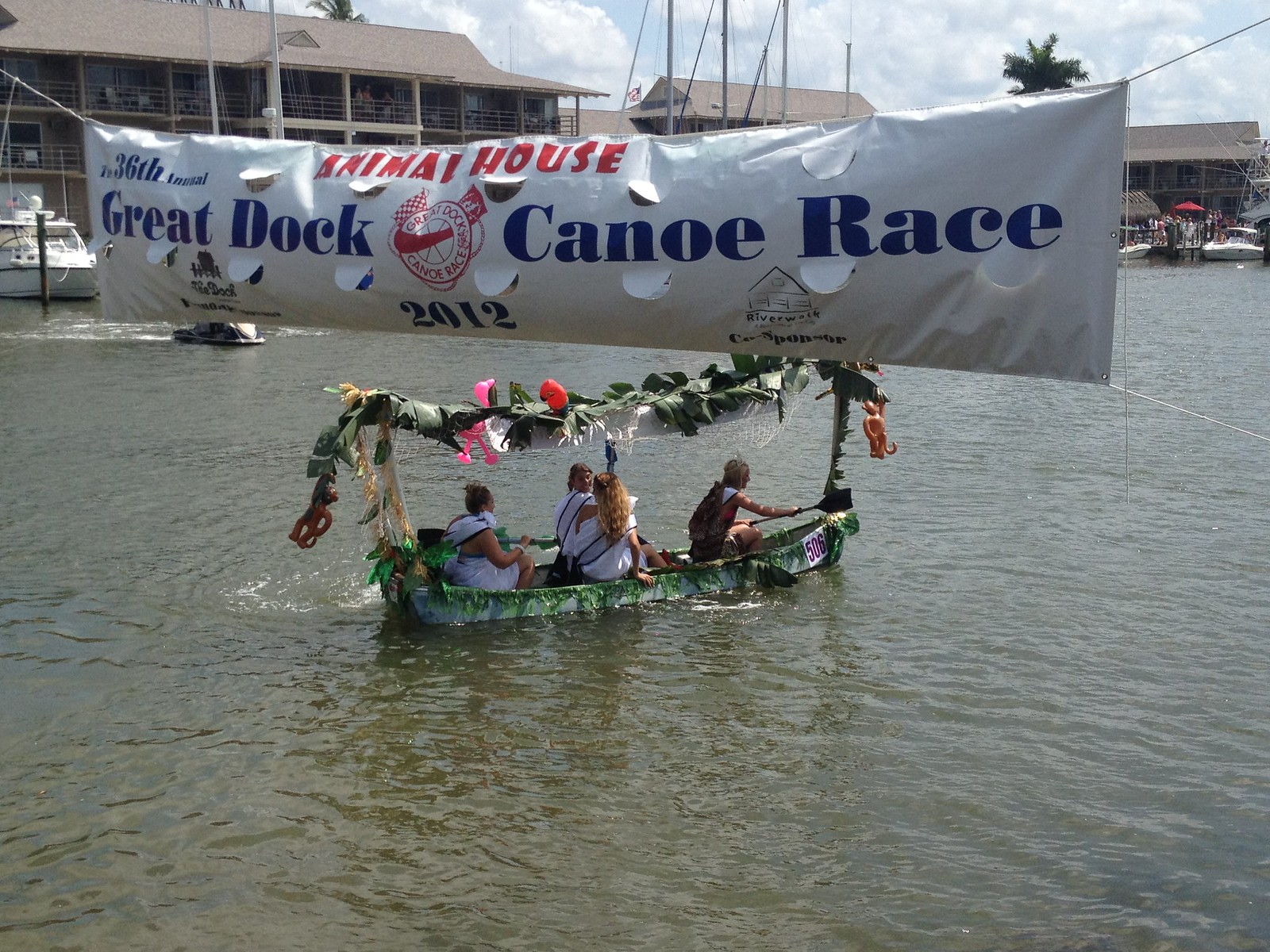In this vibrant and detailed scene, a small canoe glides across dark waters, its occupants participating in the 36th annual Great Dock Canoe Race 2012. The canoe is festooned with vines, flowers, and pink and red balloons, adding to its festive appearance. Four people are aboard: a man in a black vest and white shirt at the front, holding an oar, and three women dressed in flowing white garments with blue accents. The women in the middle have long brown hair, and the lady at the back also wields an oar and has a white garment draped over her shoulder. They appear to have just crossed the finish line, marked by a large banner above, which reads "Animal House Great Dock Canoe Race 2012." In the distance, the sky is scattered with clouds, and the backdrop features buildings, poles, boats, and umbrellas in red and white, contributing to the scene's lively atmosphere.